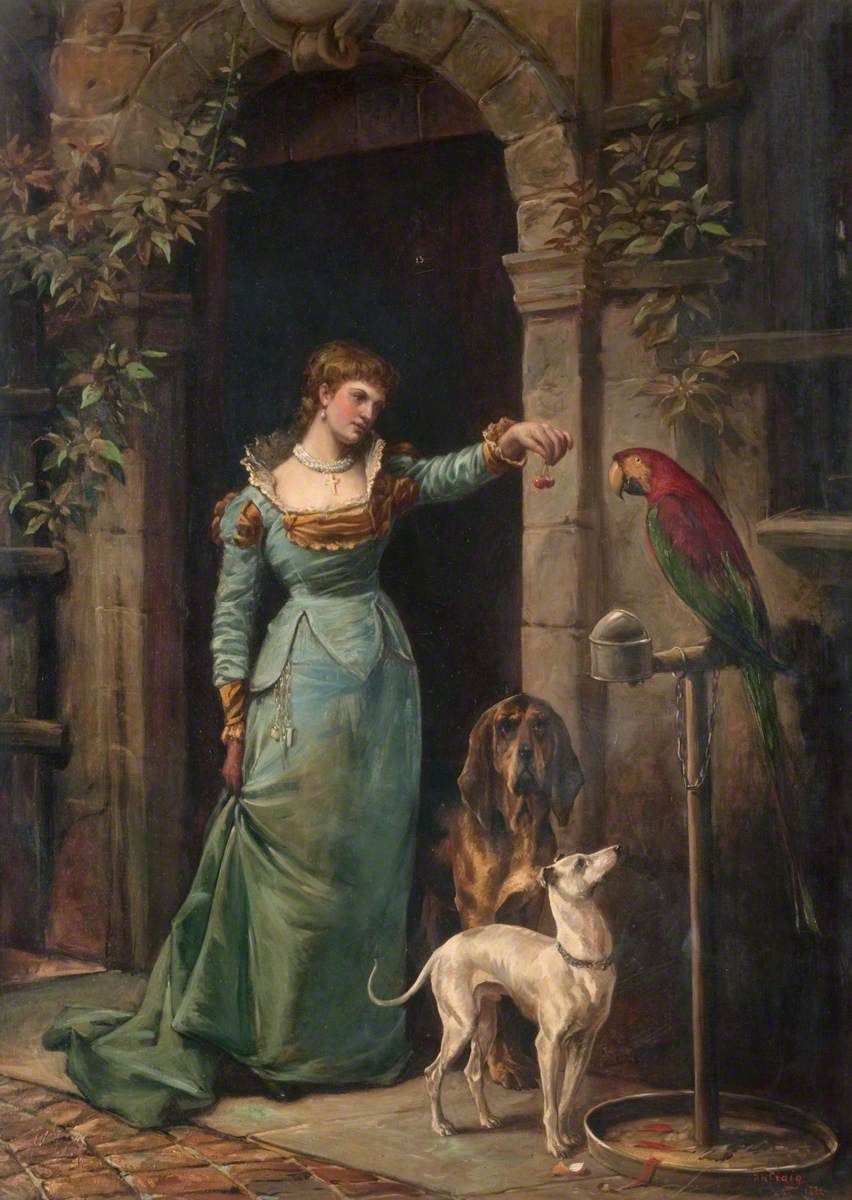This image is a detailed painting set in the early 1800s style, featuring a woman standing in the arched stone entryway of an old building with a wooden door. She wears a blue dress adorned with gold accents and full-length sleeves that have puffs on the shoulders and ruffles at the cuffs. Her dress is relatively straight but long, requiring her to hold part of it in one hand. The high lace collar adds to the ornate elegance of her attire. She has brown hair pulled back with bangs, and she accessorizes with pearl drop earrings and a thick pearl necklace with a gold cross pendant. 

The focal point is her left arm, outstretched with two cherries, seemingly ready to feed the red and green parrot perched on a metal stand before her. Beneath the parrot, gazing up at it, is a white greyhound with a long muzzle, short hair, ears that sort of fan out to the sides, and a grey collar. Beside her, to her left, stands a large brown dog resembling a hound, with long ears, adding to the serene yet attentive atmosphere of the scene.